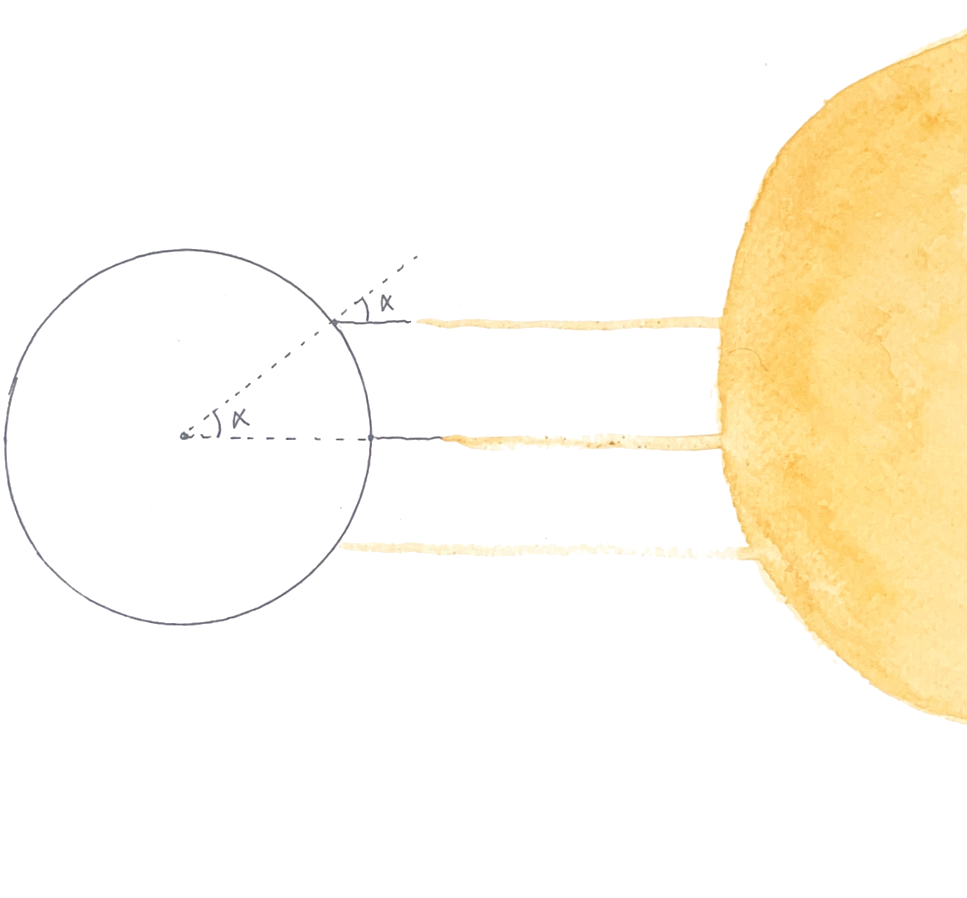The image is a detailed illustration, likely representing an astronomical concept. On the left side, there is a meticulously drawn circle, created using a pencil and a compass, with the compass points clearly visible at the center where it made contact with the paper. The circle, although neatly drawn, doesn't flawlessly meet at the starting point. Dotted black lines emanate from the circle's center, forming two radii, one extending towards the top right edge of the circle, and creating an inner angle labeled with the Greek letter alpha (α). This same angle reappears outside the circle at the intersection where one of the lines diverges.

On the right side of the image, there's a larger circle with a radiant, sunny appearance, resembling a watercolor painting characterized by its soft, yellow wash. This sunny orb generates three bright yellow rays that stretch horizontally. One of these rays intersects with the right edge of the smaller, left-side circle, highlighting the connection between the two bodies. The overlapping lines and angles suggest a mathematical demonstration, possibly illustrating the measurement of angles or the interaction of planetary bodies. The scene evokes a blend of artistic creativity and scientific precision.